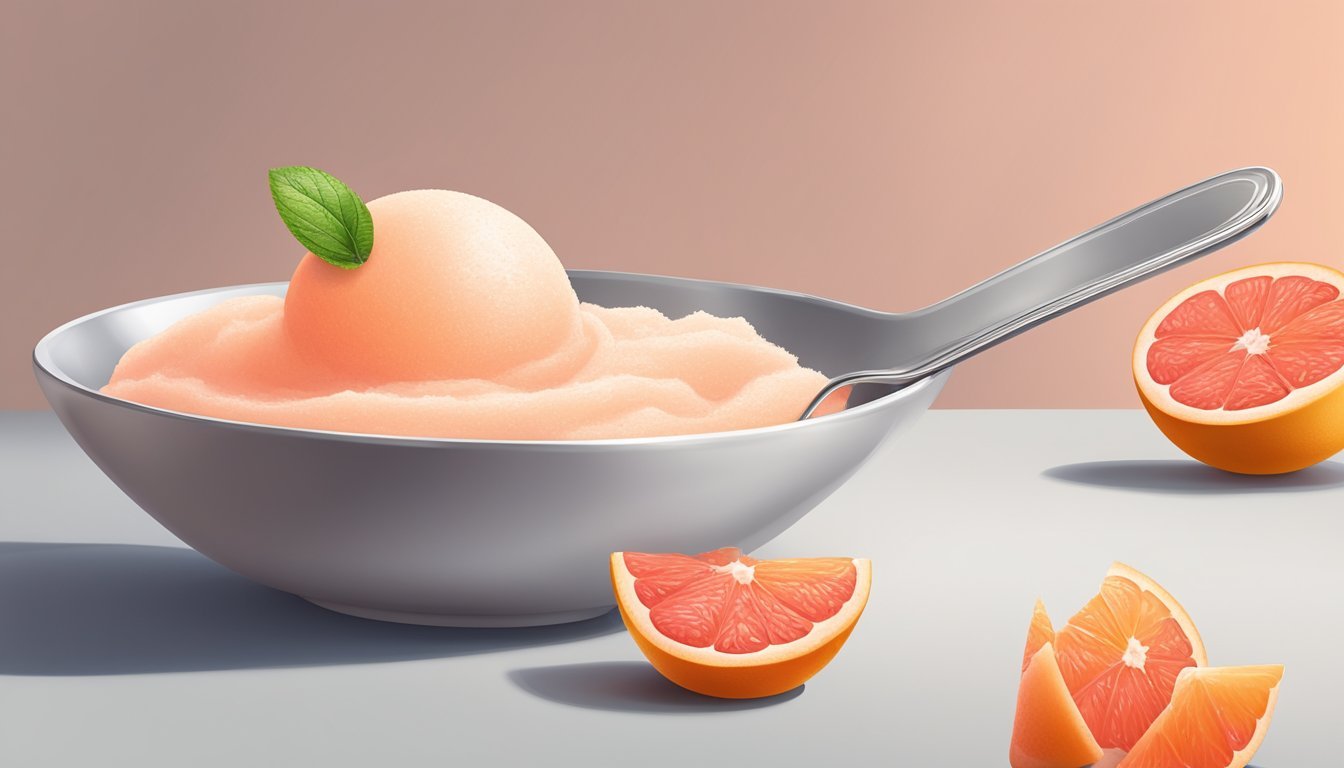This computer-generated image depicts a silver bowl sitting on a white countertop. The bowl contains what appears to be orange ice cream or sorbet, with a perfect round scoop topped by a single mint leaf. A peculiarity of the image suggests that the design might be AI-generated: a spoon or handle seems mistakenly merged into the side of the bowl. Surrounding the bowl are several orange slices, their vibrant peels contrasting with the reddish-orange, pulpy interior, reminiscent of blood oranges. The background is a muted grayish-pink, enhancing the focus on the vibrant contents of the bowl.